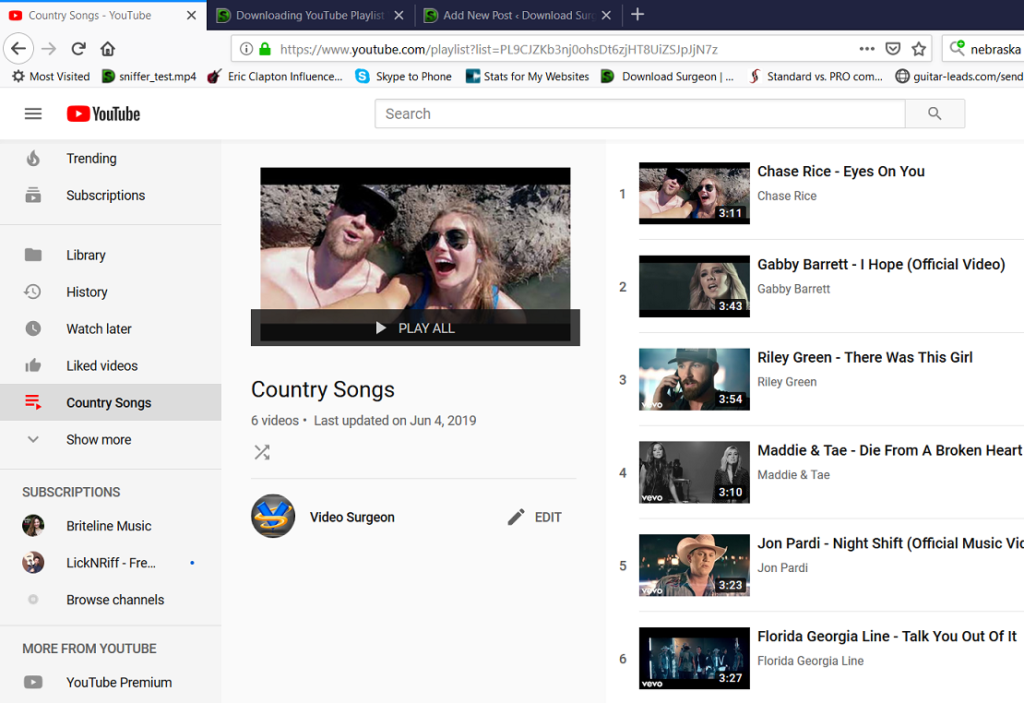Title: Country Song Playlist on YouTube

Description: This image shows a YouTube webpage displaying a playlist titled "Country Song." The playlist name is prominently displayed in the top left corner. 

**Left Sidebar:** 
- The YouTube sidebar is visible, featuring menu options such as "Trending," "Subscriptions," "Library," "History," "Watch Later," and "Liked Videos."
- There is also a "Show more" option under the Subscriptions section.
- The user is subscribed to channels including Pretty Line Music, Lick and Riff, and Browser Channels.
- At the bottom of the sidebar, it mentions "More from YouTube" and "YouTube Premium."

**Main Content:** 
- At the top of the main page on the right side, the playlist title "Country Songs" is displayed. The playlist contains 6 videos and was last updated on June 4, 2019.
- Below the update information, there is an icon with the initials "VS," where "V" is blue and "S" is yellow, representing the user "Video Sajan."
- Above the playlist details, there is a thumbnail image of a male and female taking a selfie, which likely corresponds to the first song in the playlist. A "Play All" button is also available.
- The playlist includes the following six videos:
  1. "Eyes On You" by Chase Rice
  2. "I Hope" by Gabby Barrett
  3. "There Was This Girl" by Riley Green
  4. "Die From A Broken Heart" by Maddie & Tae
  5. "Night Shift" by Jon Pardi
  6. "Talk You Out Of It" by Florida Georgia Line